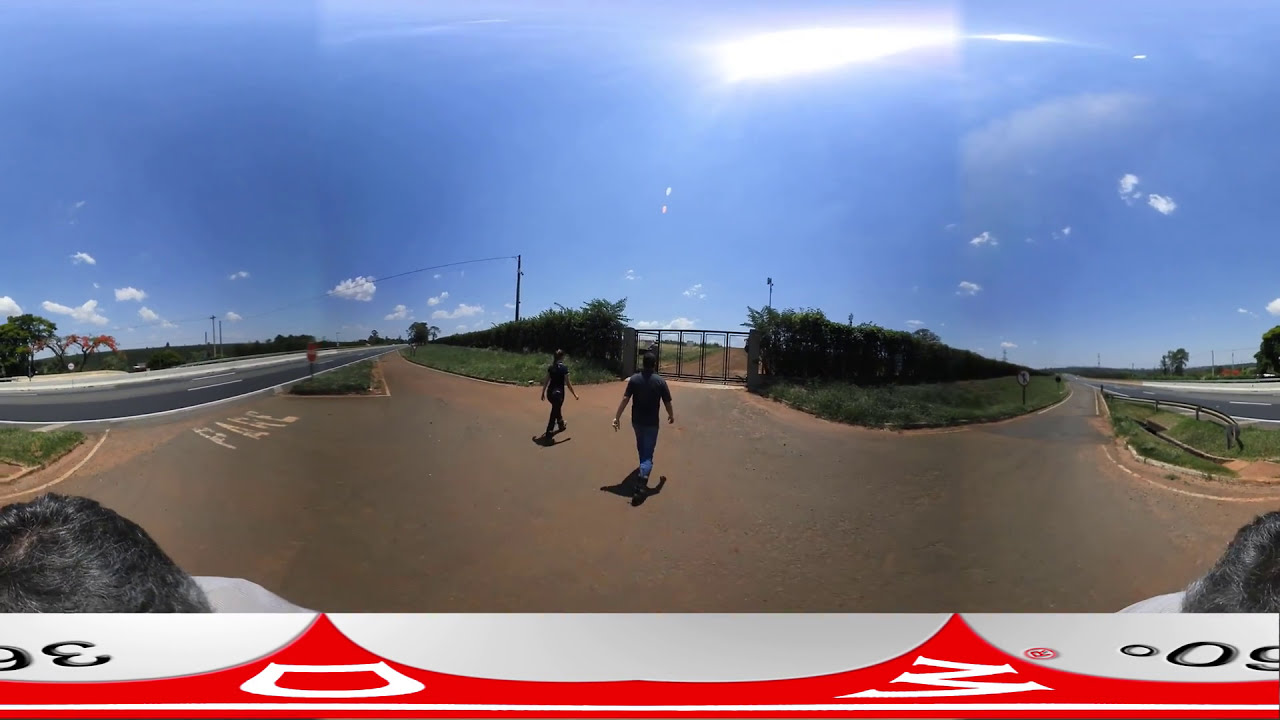In broad daylight, two people—one man on the right and a woman on the left—are walking toward a large metal gate that opens into a grassy field, which appears to be part of a park. Both individuals are dressed in green shirts and pants, suggesting they are in uniform. They walk on the right side of a two-lane road, with empty roadways on either side of them. Surrounding the road are green grass and well-maintained hedges. The bright blue sky, adorned with sporadic white clouds, and the visible sun at the top center of the image cast the scene in vivid daylight. In the bottom corners of the image, two salt-and-pepper-haired heads are barely visible, one in a white shirt. The gate ahead, positioned within the hedgerow, marks the boundary of the parking lot or park area. Red arrows and gray lettering reading "36 degrees" on the left and "6 degrees" on the right add additional elements to the bottom of the image, pointing towards the walking pair, further emphasizing the direction of their movement.